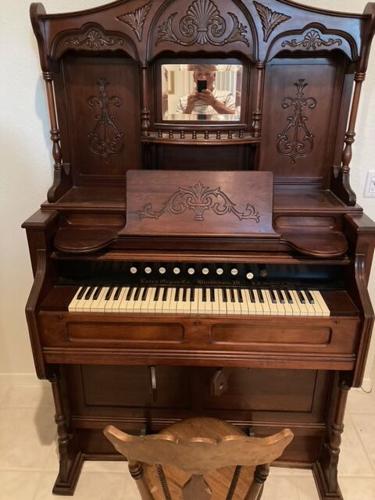The photograph depicts a beautifully ornate, antique piano crafted from dark cherry wood. The piano features intricate, decorative carvings along the top and sides, resembling shell-like and swirly curl designs. This grand piece, standing approximately eight feet tall, sits against beige walls and tile floors. A matching wooden chair, though slightly lighter and less ornate, is positioned directly in front of the keyboard. The piano keys are traditional white with black tips, and there appears to be a foot pedal underneath. Prominently displayed above the keys is a small, shiny golden plate that doubles as a mirror. In this mirror, the reflection of a person with light skin can be seen holding a cell phone, capturing the image of the piano.